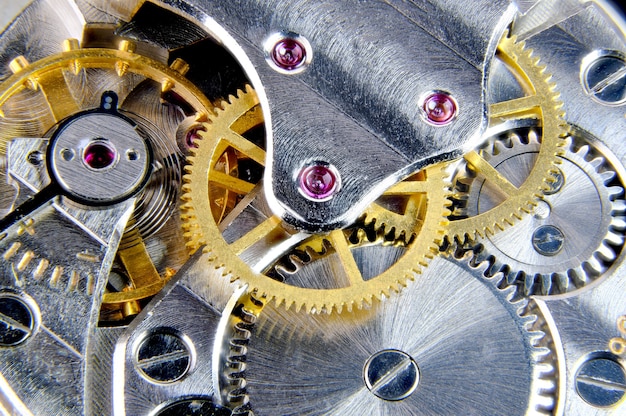This meticulously detailed photograph showcases the intricate inner mechanisms of a timepiece, likely a watch or clock. At the heart of this complex apparatus are numerous interlocking gears, predominantly gold with striking hollow interiors, complemented by a selection of silver gears. The entire mechanism is crafted from metal, accentuated by the sharp reflections of a well-lit environment. Scattered throughout are various flathead screws, their uniform design hinting at the precision engineering involved. The gears form a mesmerizing network; some are visibly engaged and intertwined, while others appear disconnected, yet integral to the overall functionality. This image captures both the artistry and technical prowess inherent in horology.